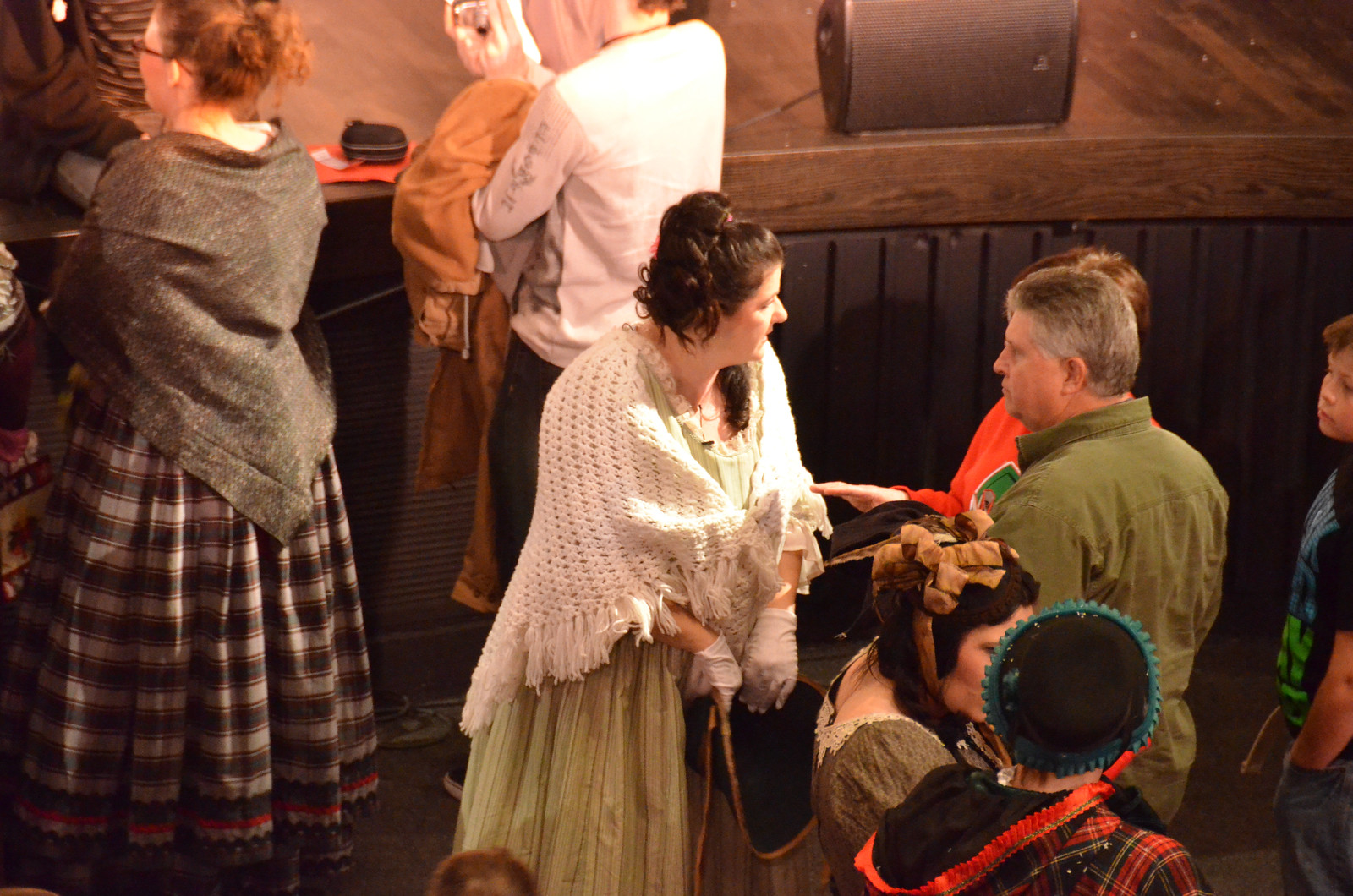This full-color photograph, taken indoors, captures a scene that appears to be either a historical event or a play set on a stage. Dominating the center of the image are a woman and a man engaged in conversation. The woman, showcasing period costume, has brown hair styled in a poofy ponytail and attire that includes white gloves, a white knitted poncho over a green dress, and she holds an old-fashioned purse. Behind her, another woman sports historical ribbon headgear and a dress reflecting an older style. The man she is talking to appears to be in his late 40s or early 50s, with salt-and-pepper gray hair, and is wearing a green shirt, which may be short-sleeved but is partially cut off in the photo. The background includes several other individuals clad in similarly old-style clothing, as well as a young boy positioned near an older man. The image also features wooden walls, some painted, a dark-colored ground surface possibly covered in carpeting or tile, and overhead speakers. No text indicating names, dates, or location is present, and the multitude of colors in the image includes black, white, red, orange, green, blue, and brown.